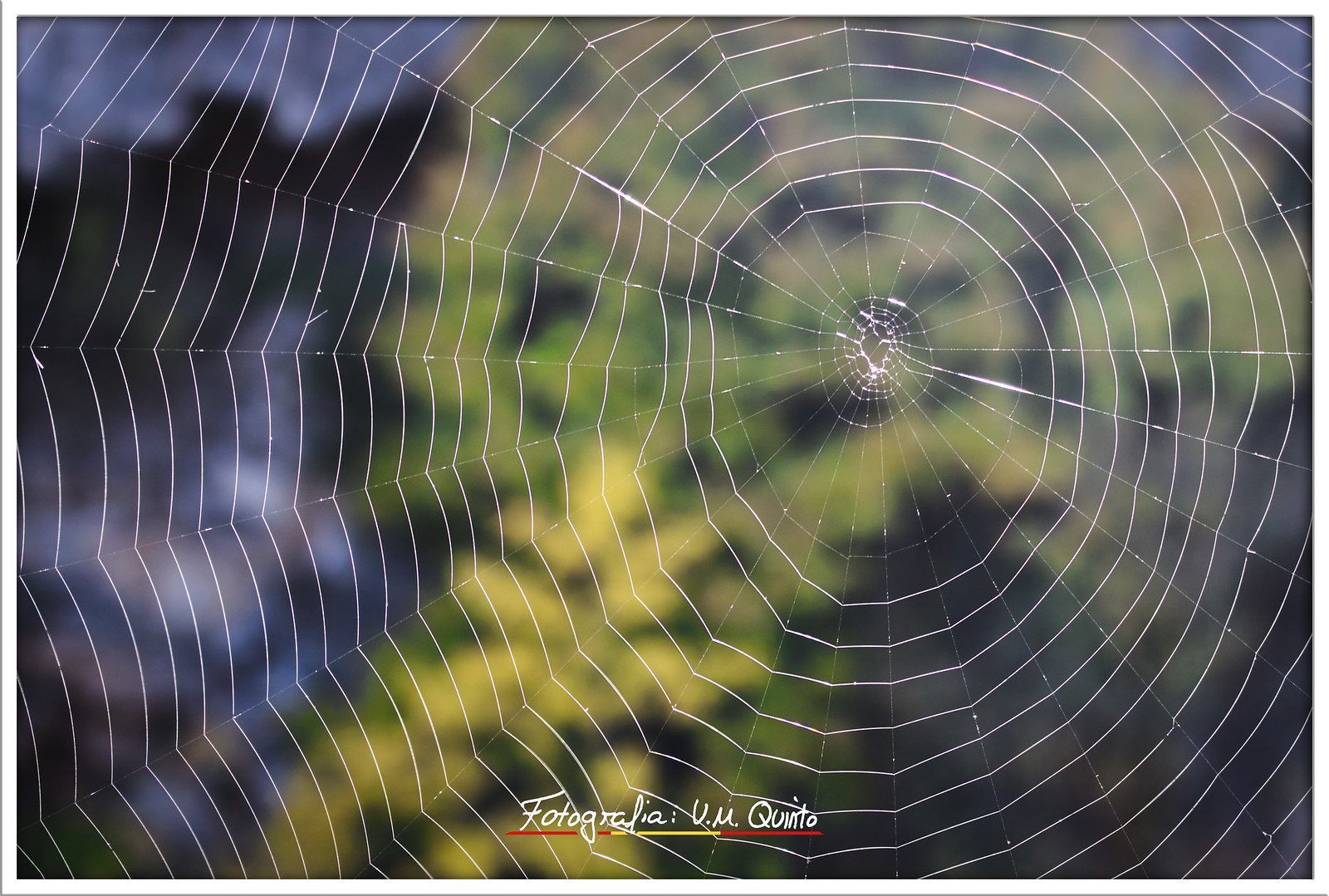The image captures a beautifully intricate spider web positioned slightly off-center towards the right. The web is meticulously organized, almost perfectly circular, and spans a large area, extending all the way to the left and beyond the frame. The delicate, white threads of the web are finely detailed, appearing almost like lacework. Behind the web, the background is artistically blurred, but hints of green near the center and darker blue shades further out suggest the presence of a tree or foliage. At the bottom of the image, the text "Fotografia UM Quinto" stands out in white, underlined with a red and yellow line, adding a touch of artistic flair to the composition.